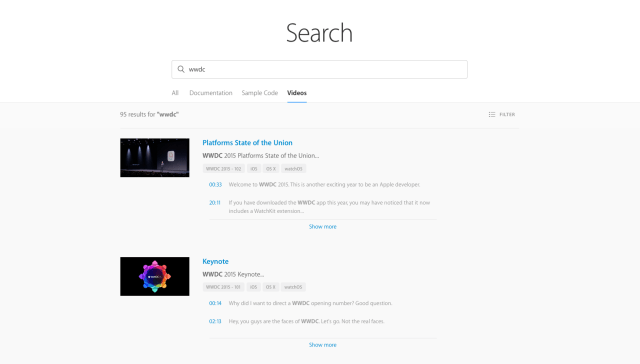The image depicts a search interface on a website with a white background. The search results are for "WWDC platform, State of the Union." Specifically, it shows 95 results, including notable entries such as "WWDC 2015 platform, State of the Union" and "WWDC 2005 Keynote." There is a blue underline beneath the word "videos." Additionally, there are options to "Show more" and "Filter." The image indicates there's more information available in the description. A call-to-action in Spanish at the bottom reads, "¡Vamos al vídeo!" suggesting the viewer should watch the associated video content.